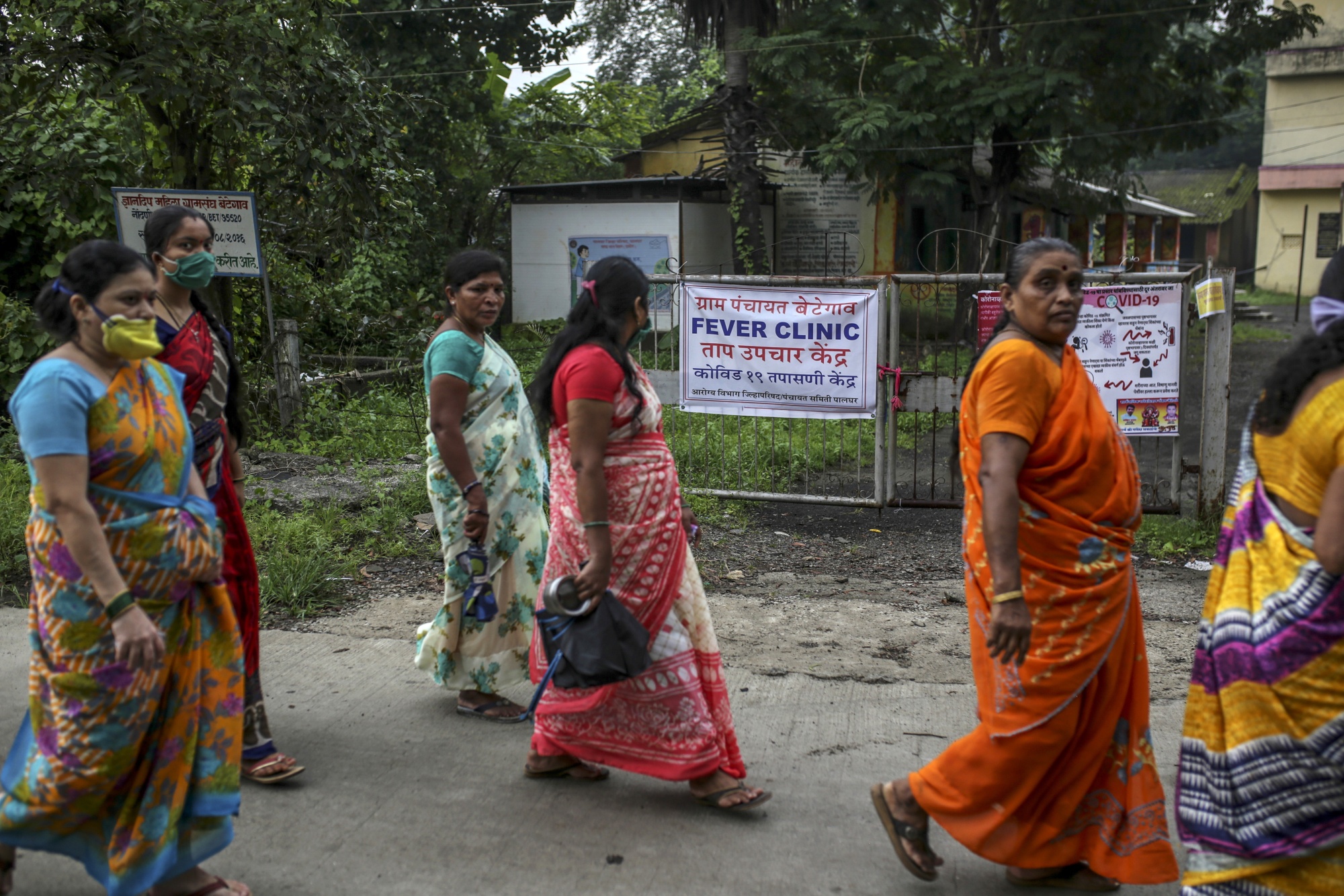The image captures six Indian women walking from left to right on a concrete path, presumably heading towards a fever clinic. A fence in the background prominently displays a white sign with blue text that reads "Fever Clinic," accompanied by information about COVID-19. Behind the fence, yellowish, possibly rundown buildings with red awnings and pillars are nestled among trees and other greenery, indicating a somewhat rural setting.

The women are dressed in vibrant, traditional saris, each adorned in a unique combination of colors, including yellows, oranges, reds, blues, and purples. Their outfits are draped gracefully, reflecting their cultural heritage. Some of the women have masks on, likely due to the pandemic, with the two women at the back wearing masks—one in a yellow mask below her nose, and the other in a green mask. 

At least three of the women are looking towards the camera, although not with particularly happy expressions, while others are either looking away or have their faces turned in different directions. Detailed attire descriptions include a woman in a yellow and purple sari, another in an orange sari with a blue and yellow embellishment, one in red and white, and another in teal and cream. Their dark hair is styled in various ways, either pulled back or partly clipped up. The scene suggests a mix of anticipation and solemnity as they make their way to what appears to be a clinic amid the ongoing health crisis.